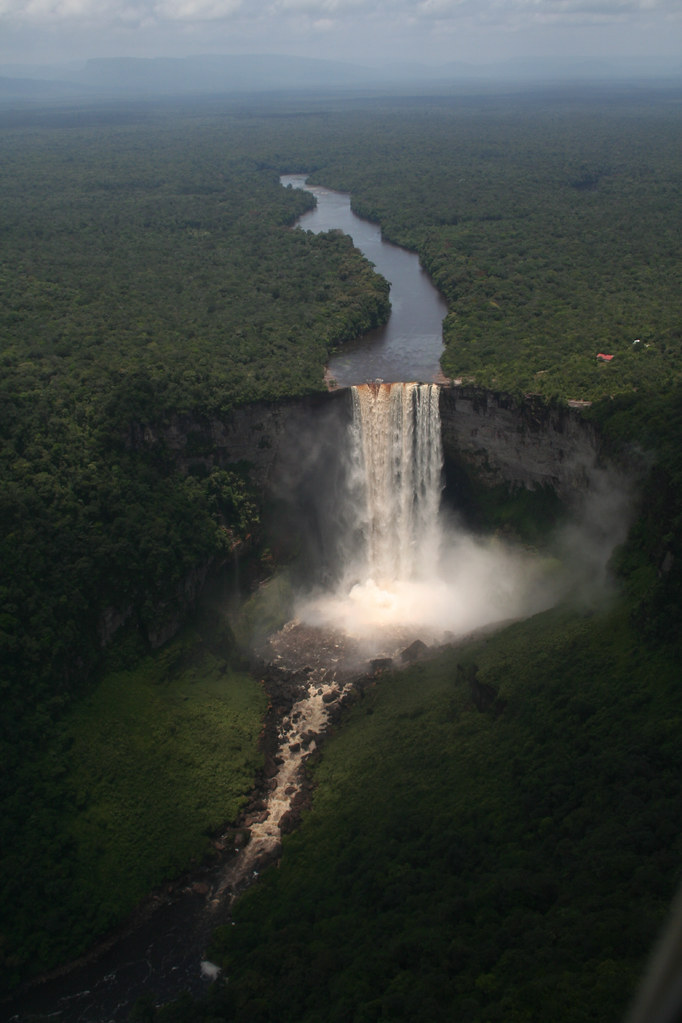This is a breathtaking aerial photograph of Kayator Falls, showcasing its majestic beauty. At the center, a massive waterfall cascades from a towering cliff into a large reservoir below. From there, the water meanders into a small stream that flows downhill toward the bottom left corner of the image. The waterfall is nourished by a river above, which winds through dense, lush jungle visible on both sides of the photograph. The landscape is enveloped in verdant greenery, with abundant trees and rocky cliffs adding to the natural splendor. In the background, a hazy mountain range looms, partially obscured by fog and distant clouds. A small building perches on the right side of the waterfall atop the mountainous terrain, overseeing the verdant valley that gently slopes around the river. The overall scene is a testament to the astonishing beauty and natural wonder of our world.